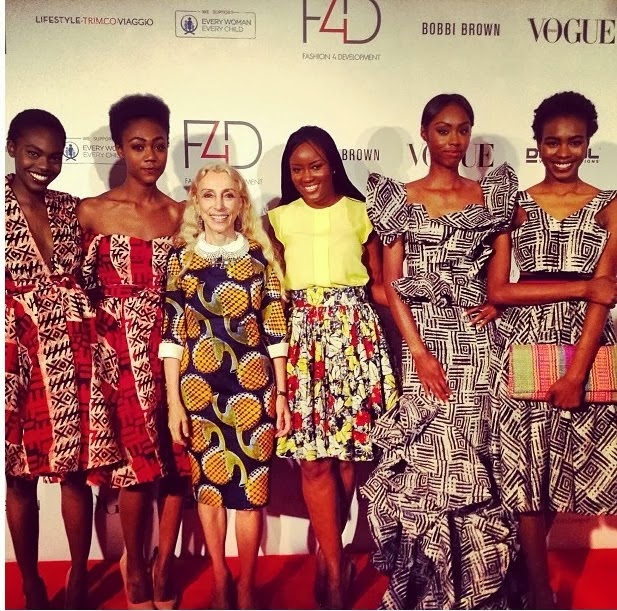The photograph captures six elegantly dressed women posing on a red carpet. Among them, five are African-American and one is a Caucasian woman. The backdrop displays prominent fashion-related brands, including "Vogue" and "Bobby Brown," suggesting a high-profile event. The group exhibits a mix of coordinated and unique styles, reflecting a fashion showcase.

On the far left, two African-American women are adorned in matching dresses with red, black, and white stripes. The dresses have distinct shoulder designs; one is shoulderless, while the other covers the shoulders. The woman on the far left is smiling with her teeth, showcasing her shorter black hair, whereas the next woman has a neutral expression and very short hair.

Standing centrally, the Caucasian woman sports a dress with a vibrant pineapple print on a black background. She is smiling brightly and has long blonde hair. Next to her, an African-American woman is glowing in a yellow top and a long, flowery skirt. She has long hair and is also smiling with her teeth.

On the right side of the image, two African-American women wear dresses featuring a black and white pattern, albeit in different styles. One has a shorter dress with shorter sleeves, while the other dons a longer dress with poofier sleeves. The woman on the far right is holding a pink and green clutch and has her hair tied up, smiling, while her counterpart has short hair and is smiling with her teeth.

The entire scene is set against a white backdrop adorned with the text "Vogue" and "Bobby Brown," emphasizing the fashion-forward and glamorous nature of the event. The women’s coordinated yet distinct styles, their confident expressions, and the vibrant setting collectively create a striking tableau of contemporary fashion.